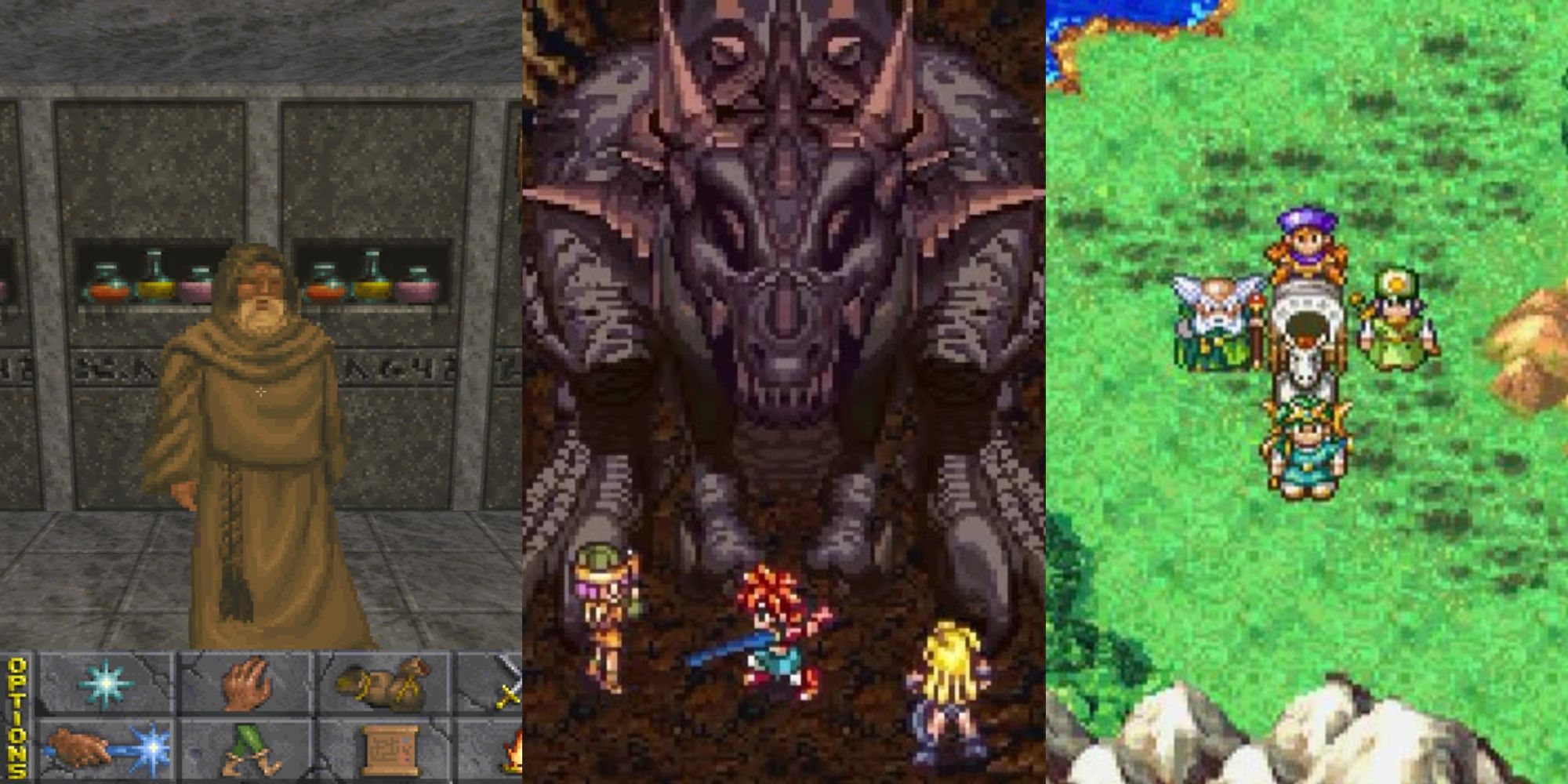This composite image is a screenshot from an 8-bit video game, divided into three distinct sections. On the left side, a medieval-styled merchant, donned in a brown robe with a rope belt and a hood, stands inside a gray-walled shop. Behind him are shelves lined with potions. The bottom of this section displays clickable options and icons like hands, feet, and swords, indicative of an in-game purchasing interface.

The center section showcases a dramatic scene featuring a large, demon-like creature with multiple horns protruding from its head, colored in dark bronze, dark brown, and dark gray shades. The creature, with its imposing jaw and sharp white teeth, dominates the screen. Below it are three small 8-bit characters, each distinctly dressed: one with blonde hair, another with red hair wielding a long blue sword poised to attack the demon, and a third character wearing a green helmet.

On the right side of the composite image, a peaceful green grassy field scene reveals four 8-bit characters encircling a horse-drawn wagon, with a water body visible in the background. The entire image maintains a pixelated aesthetic reminiscent of 1990s video games.